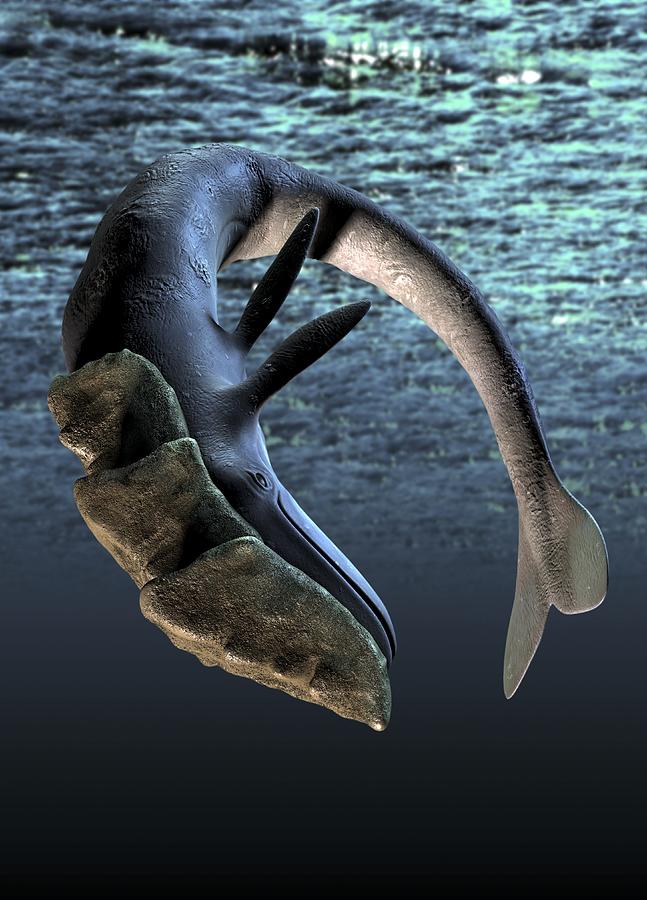The image is a rectangular photograph, approximately six inches in height and four inches in width. The top half of the background depicts shallow water, rendered in shades of green and gray, creating the impression of an approaching shoreline, although the shoreline itself is not visible. The bottom half of the image transitions from a dark gray to an almost black gradient as it progresses downward.

In the center of the image, there is a model of a prehistoric whale in a dynamic diving pose. The whale's head, which features three large, brown bony plates, points downward while its arched back curves gracefully upward and then back down, bringing the tail almost level with the head. The whale's back is a darker gray, while its underbelly is a lighter gray. It has a long snout, a small eye, and two elongated paddle fins positioned on its sides. Notably, the whale lacks a dorsal fin. Its tail splits into two rounded fins, completing the detailed representation of this ancient creature.